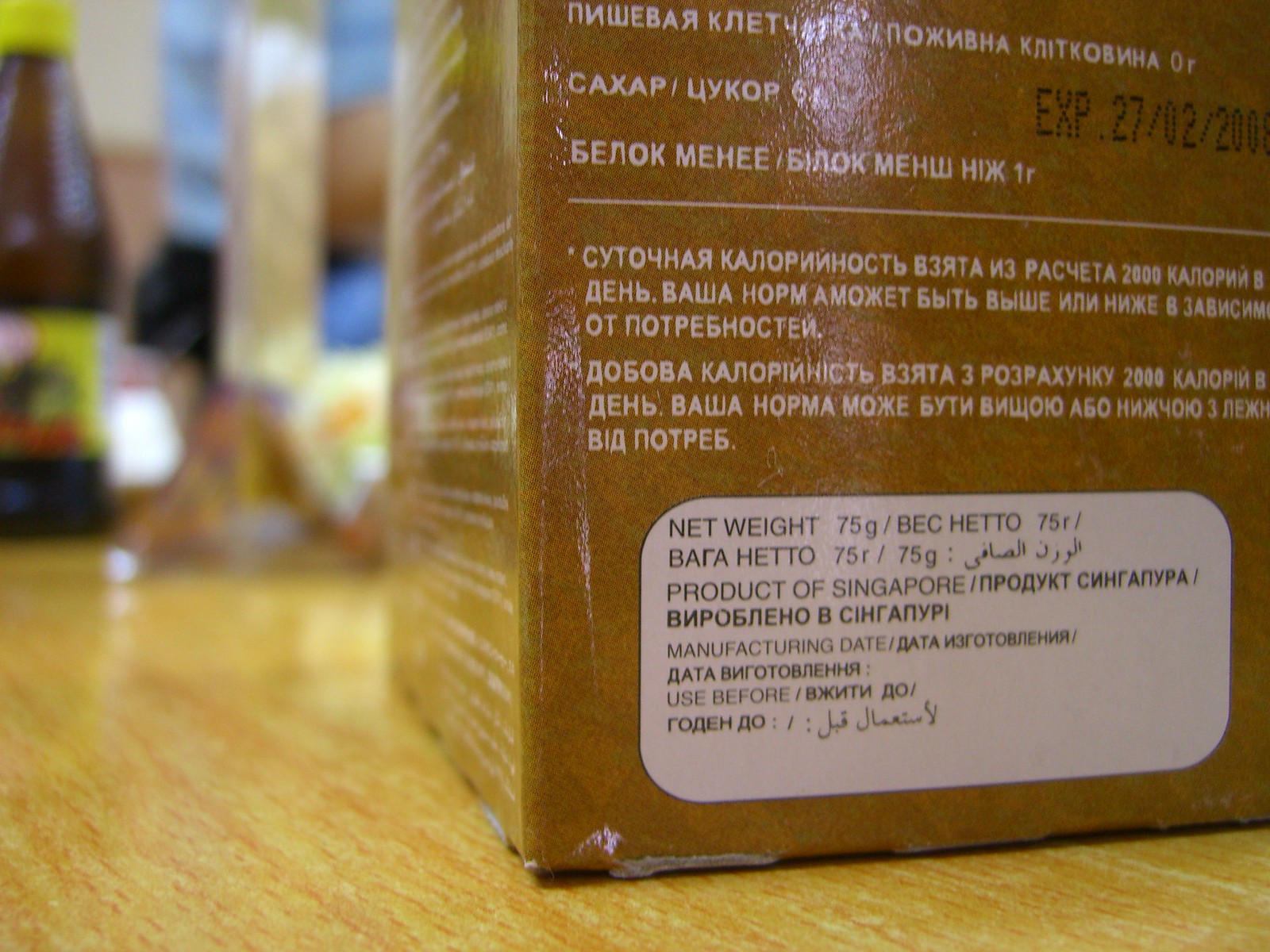The image features a food item in a light brownish carton with white foreign lettering, primarily not in English. The net weight of the product is indicated as 75 grams. The packaging displays both a manufacturing date and a "use before" date; however, the "use before" date is listed in a different language. Notably, the expiration date on the side of the box reads February 27, 2008. This product is identified as originating from Singapore. The box is placed on a wooden table, providing a rustic backdrop to the scene.